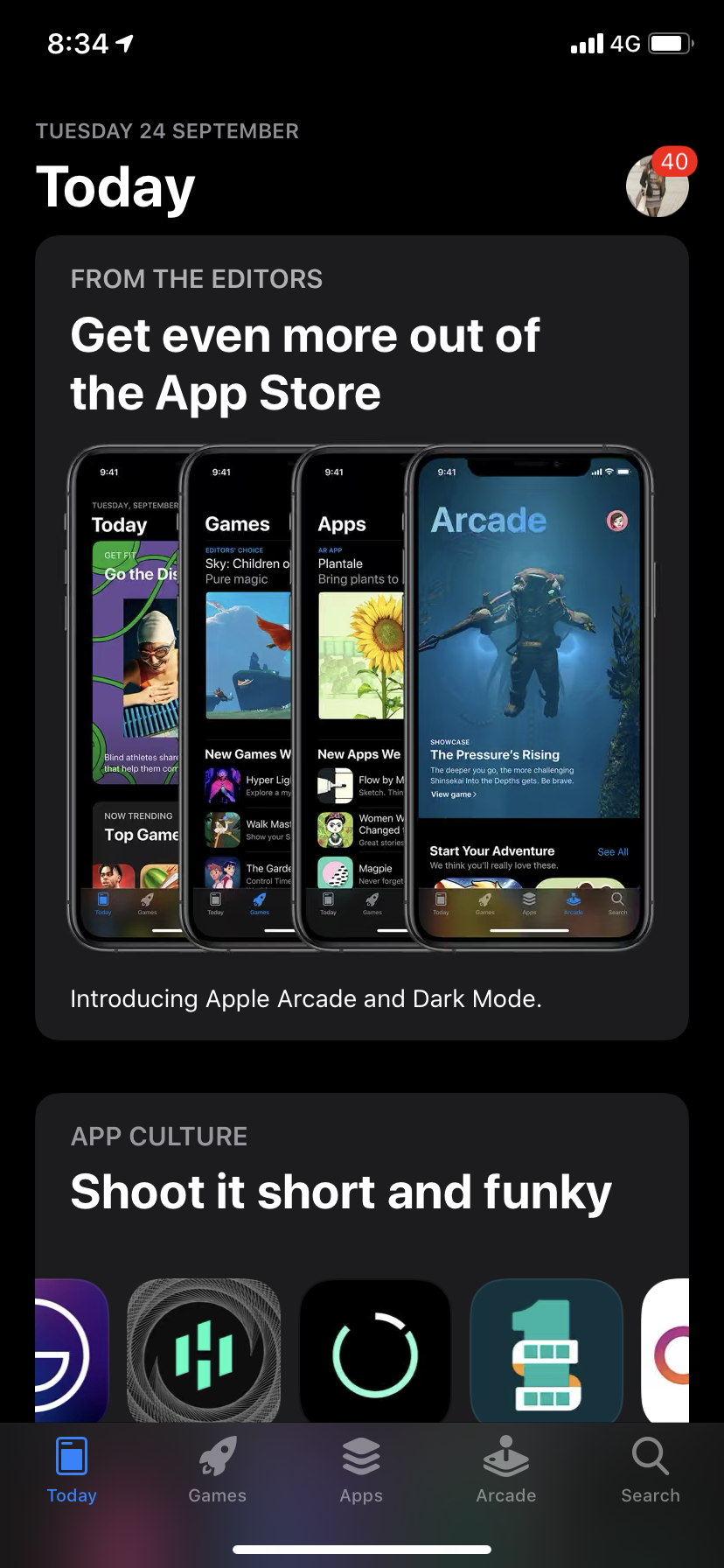The image displays a smartphone screen with full bars of 4G connectivity and a battery level at 75%. The date shown is Tuesday, 24 September. The top section includes a profile picture featuring the number 40 in red. The central part of the screen highlights a notification from "the editors," encouraging users to get more out of the App Store.

The visual theme includes four illustrated phones stacked vertically, each depicting different graphics: a man in swimwear, an animated boat, a yellow sunflower, and a scuba diver. A promotional message reads, "The pressure's rising. Start your adventure." Additionally, it introduces Apple Arcade alongside the Dark Mode feature.

A variety of app icons are displayed, emphasizing the dynamic nature of app culture with the tagline, "Shoot it short and funky." Tabs at the bottom of the screen indicate different sections of the App Store: Today, Games, Apps, Arcade, and Search. A navigation line is visible at the bottom, indicating the currently selected tab.